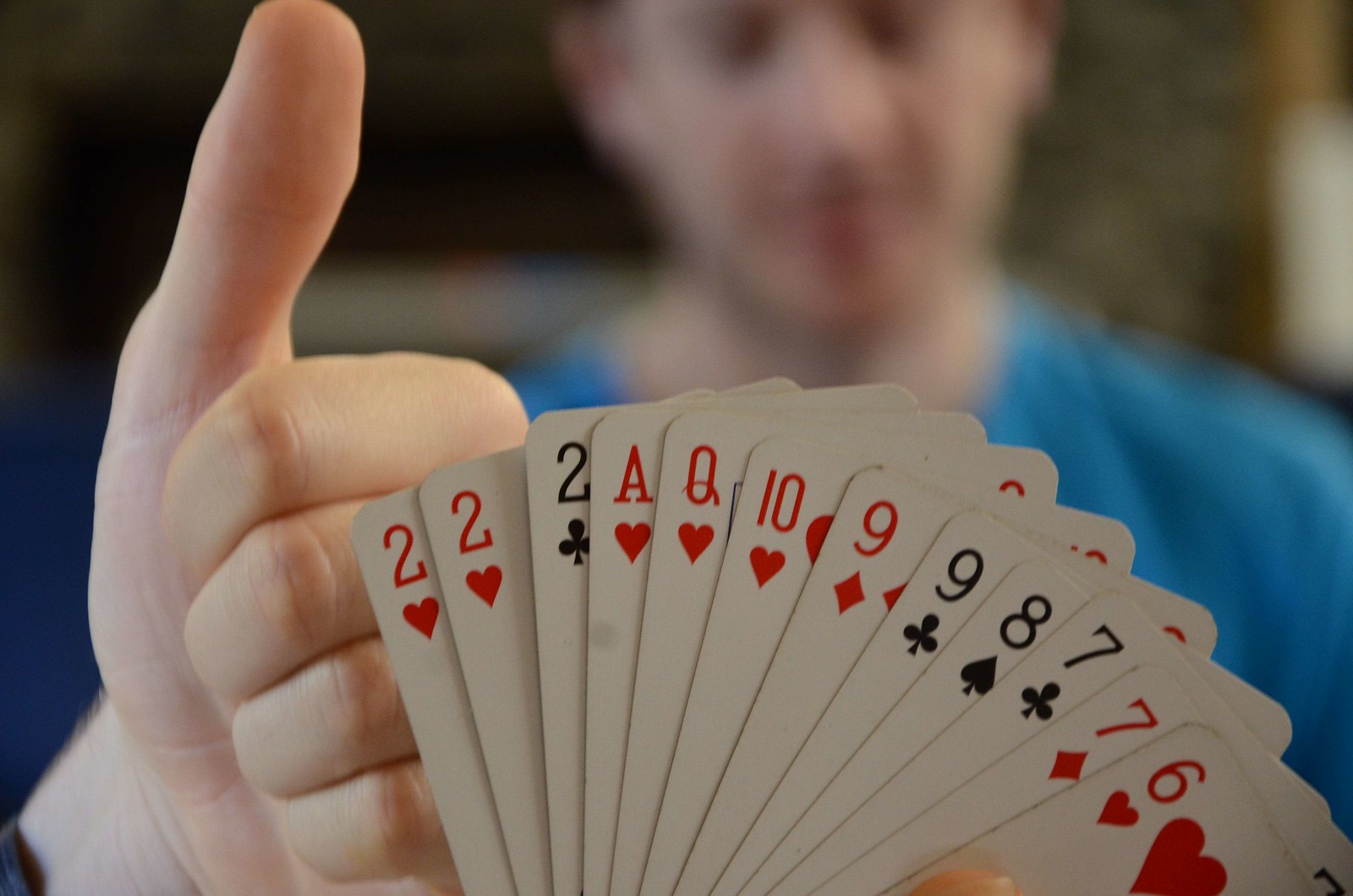A person is holding up a deck of standard playing cards prominently in the foreground of the image. The cards displayed from left to right include: two of hearts, two of hearts, two of clubs, ace of hearts (which has a noticeable stain), queen of hearts, ten of hearts, nine of diamonds, nine of clubs, eight of spades, seven of clubs, seven of diamonds, and six of hearts. The cards are all white with red and black writing. In the background, a blurry Caucasian man can be seen wearing a white and blue shirt. To the top left of the image, another hand is making a thumbs-up gesture. The background itself features a wall with a mixture of black and off-gray colors.